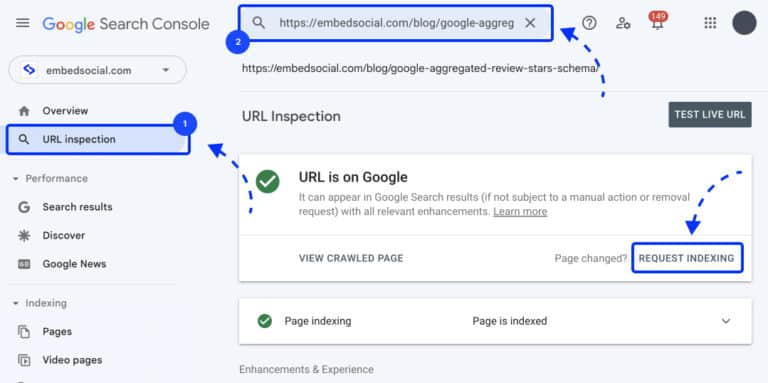A detailed caption for the described image could be:

---

A screenshot of a webpage from embedsocial.com, specifically the blog post "Google Aggregated Reviews Star Schema," is displayed. The main interface is Google Search Console, even though the background is light gray and the URL indicates it's on EmbedSocial’s website. On the left pane, various sections are visible, including Overview, URL Inspection, Performance (with subsections like Search Results, Discovery, Google News), and Indexing (with visible submenus like Pages, View Pages). The central section is focused on the URL Inspection tool, with a highlighted indication that the URL is on Google and can appear in search results with all relevant enhancements. Specific elements in the image are annotated with numbered labels: "1" highlights the URL Inspection tool, and "2" emphasizes the address input field and the "Request Indexing" button near the settings icon. This interface is crucial for assisting in the identification and indexing of web pages by Google.